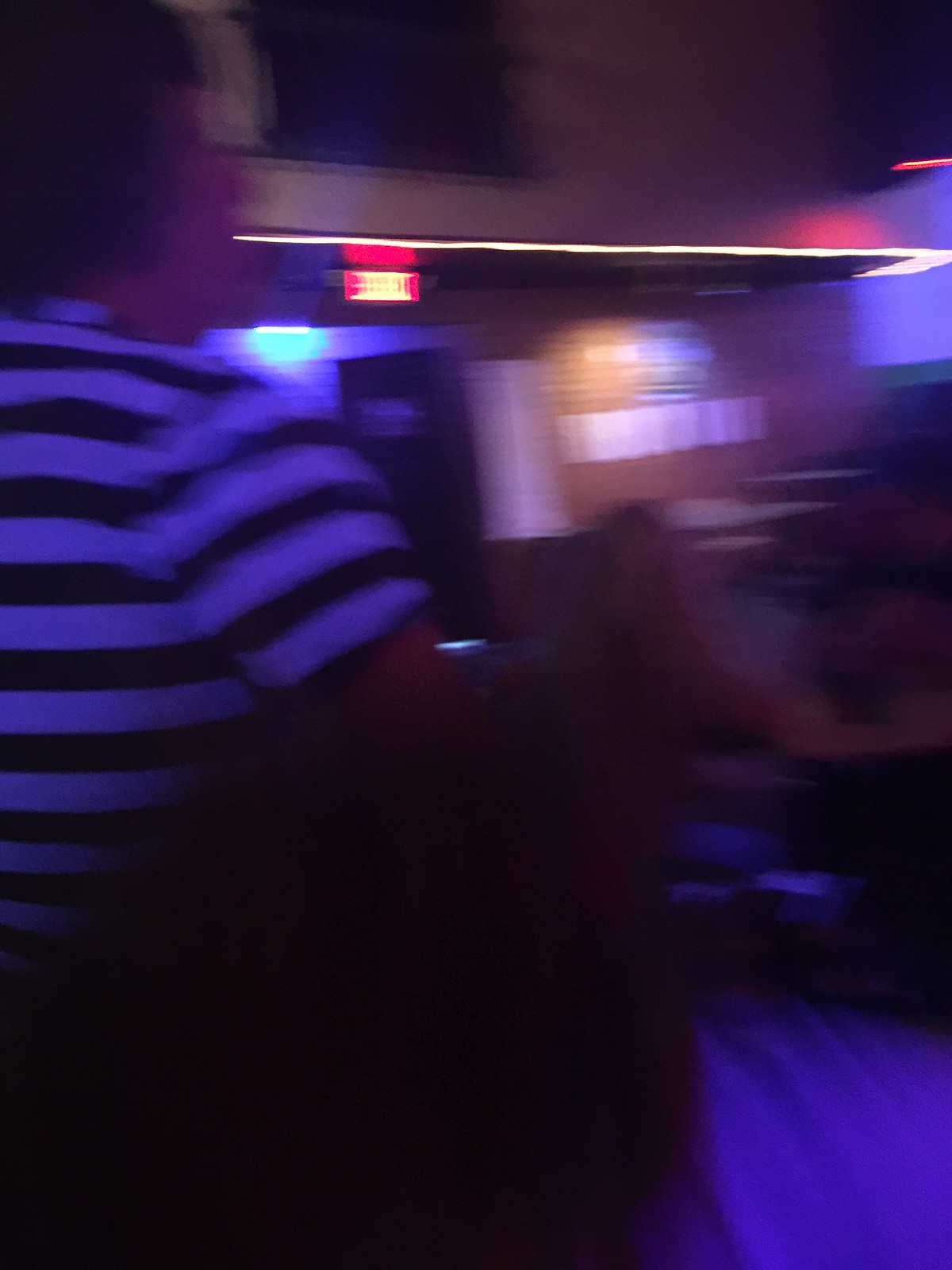In a dimly lit room with a warm, brownish-red hue, a person wearing a white and black striped shirt stands prominently. The individual, who has short hair and may be wearing glasses, faces two others seated at a table in front of them. One of the seated individuals has long blonde hair, while the other sports a black t-shirt and short black hair. The table where they sit is among several others scattered in the background, suggesting a communal or meeting space within the building.

Illumination in the room comes from a variety of light sources: a bright white light, a blue light, a long fluorescent white light, and a square red light. The walls bear several white papers, possibly notices or posters, creating a subtle contrast against their reddish-brown surface. To the left, there is a white door and beside it, a brown door, adding to the room’s eclectic decor. 

On the right side of the wall hangs a white projection screen, and above the lights and doors is a peculiar black cutout—potentially a sign—adding a mysterious element to the otherwise straightforward room. The overall scene evokes a sense of a casual, perhaps educational or collaborative, environment.